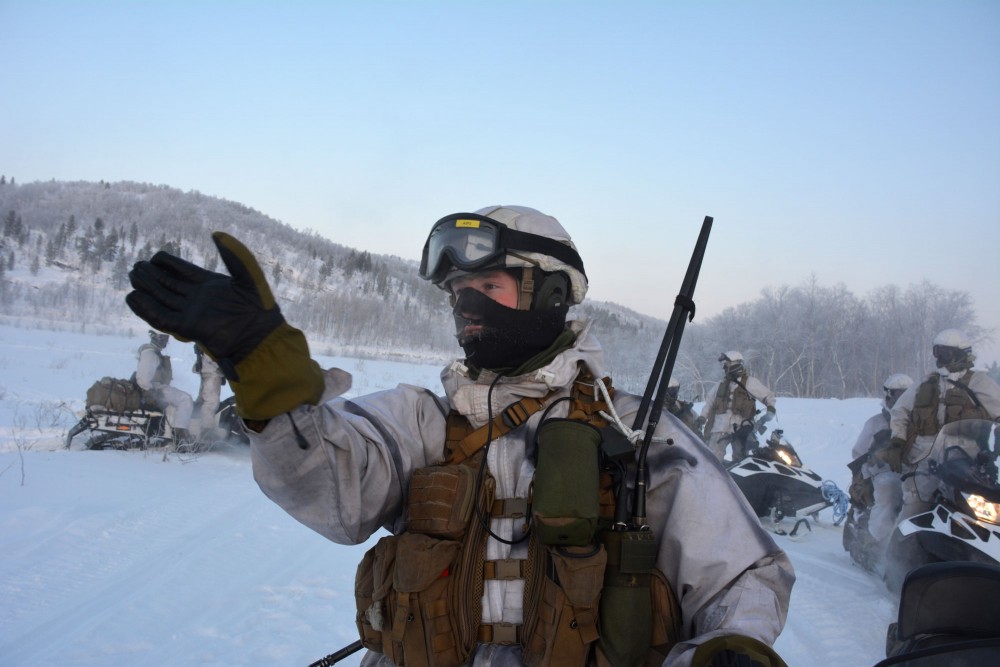In a snow-covered, wooded area, a group of men clad in beige camouflage are depicted in a hunting scenario. This photograph captures the team navigating the terrain on snowmobiles, paired in twos with each vehicle. They are equipped with essential gear including cargo bags, radios strapped to their chests, and canteens, showcasing their preparedness for the elements. The men wear protective winter attire, featuring thick dark gloves, helmets, black snow goggles, and face masks to shield against the cold. One individual stands out in a close-up, pointing into the distance with his gloved hand, possibly directing the group's attention to something in the canopy of barren and pine trees, which are all blanketed in fresh snow. The backdrop highlights the expanse of the snow-covered ground, forest, and distant snow-laden hills, reinforcing the harsh and remote environment they are traversing.